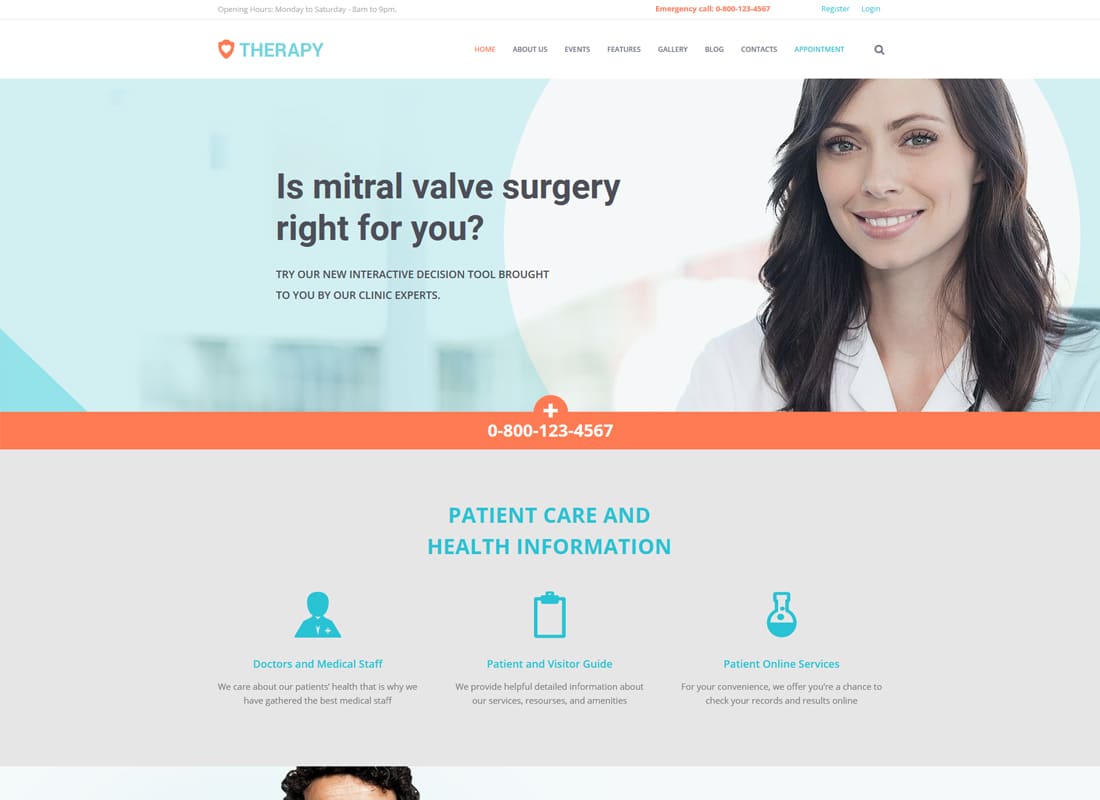Screenshot of Health Website with Detailed Information Highlighted:

The screenshot depicts a health website open on a computer. At the top of the page, it displays the opening hours: "Monday through Saturday, 8 a.m. to 9 p.m." Beneath this, the word "Therapy" is prominently shown in blue. 

To the right of "Therapy," there is a section titled "Emergency Call" followed by a phone number for immediate assistance.

A navigation bar filled with various clickable options is visible, with the "Home" button highlighted in orange, indicating the current page being viewed.

Below the navigation bar is a rectangular image. On the right side of this image, there is a young woman with long, dark hair smiling at the camera. To the left of her, in bold black text, the caption reads: "Is Mitral Valve Surgery Right for You?" Directly below this headline, smaller text invites users to "Try our new interactive decision tool brought to you by our clinic experts."

An orange bar separates this central image section from additional information below. Within this bar, the emergency phone number is repeated for easy access.

At the bottom of the screenshot, there is a gray, horizontal rectangle with categories written out in blue. From left to right, the categories are:

1. **Doctors and Medical Staff** - Depicted by an icon of a person, with subsequent gray text providing further subcategories or details.
2. **Patient and Visitor Guide** - Represented by a clipboard icon, followed by gray text with additional information.
3. **Patient Online Services** - Illustrated with a test tube icon, accompanied by gray explanatory text.

Finally, at the very bottom edge of the screenshot, there is a partial image of a person's head with dark hair, suggesting that more content is available if the user scrolls further down the page.